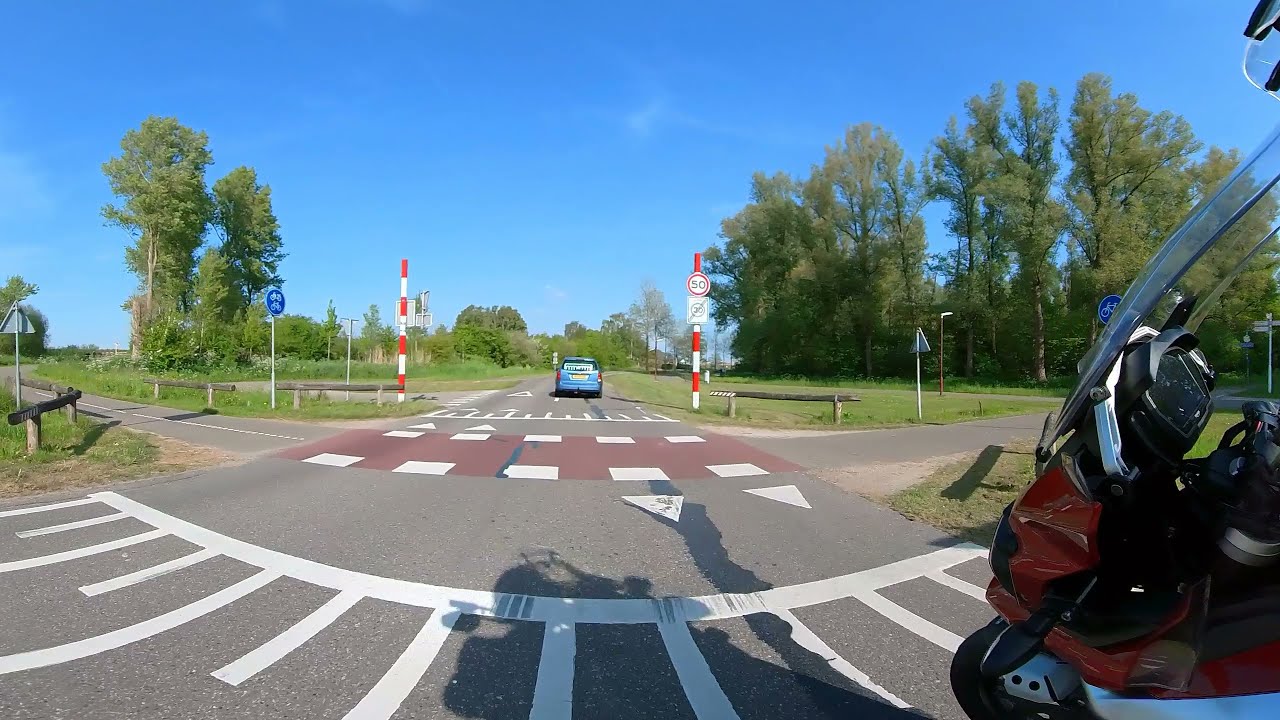The image depicts a clear, bright day in what appears to be a European setting, indicated by distinctive street signs and markings. The scene centers around a crosswalk in a small, asphalt-paved two-lane road flanked by red and white striped posts. Prominently displayed is a speed limit sign indicating "50" in a red circle. Just past the crosswalk, a blue car with a yellow back license plate is visible, having crossed an intersection intersected by a bike path. To the right, a notable red and white motorcycle or moped with a curved canopy can be seen. The background reveals numerous trees, wooden railings, and a sky that's impressively clear with only a few misty clouds, emphasizing the likelihood of it being spring or summer. The overall scene exudes a sense of a typical, peaceful day in a foreign, probably European, locale.